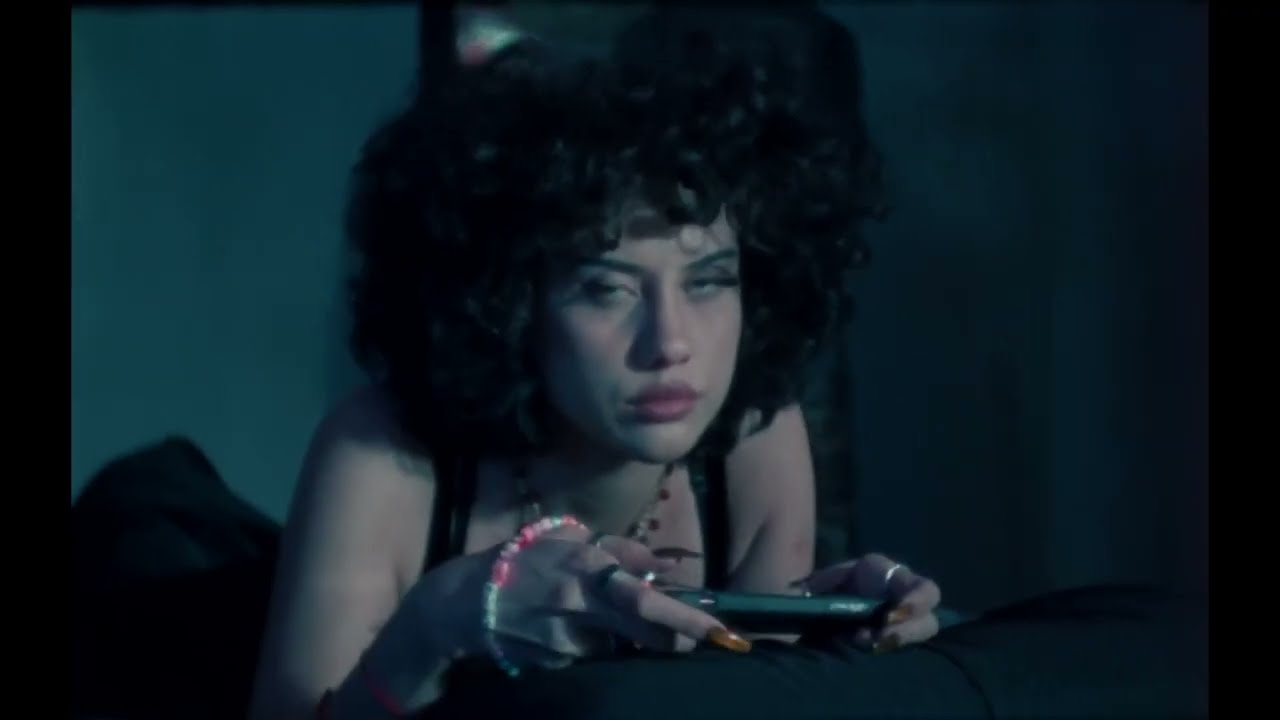In the dimly lit, almost evening-like setting, a woman with an upset or disappointed expression lies on her stomach, possibly on a bed with dark covers. She has dark, thick, poofy hair that spreads out widely across her head, reaching just above her eyebrows and covering her ears. Her Caucasian skin has a slightly dark tone, and her partially open eyes reveal brown pupils, giving her a look as if she’s rolling her eyes. Her lips are pink, adding a touch of color to her moody visage.

She wears a sleeveless, black tank top and is adorned with several pieces of jewelry: a beaded bracelet with pink and light green elements, a necklace with mostly white beads and small red dots, and rings on her index fingers of both hands—one dark and one shiny silver. Her fingernails are long and gold-colored, adding to her dramatic appearance.

In her hands, she holds a smartphone sideways, suggesting she might be playing a game. The background splits into two distinct colors with a completely dark black on the right side and a dark green hue on the left, emphasizing the contrast in the dimly lit room.